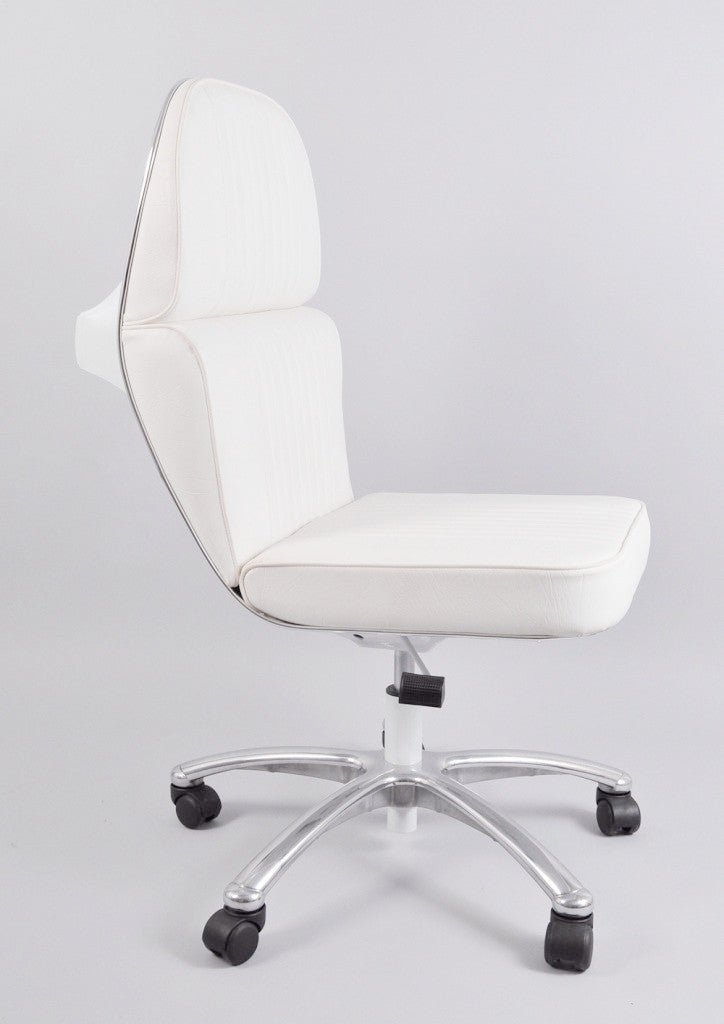The image depicts a white office chair with a padded, possibly leather or vinyl, seat and backrest, positioned against a predominantly white background that may have light gray tones. The chair's design features a segmented back cushion consisting of two parts: a lower section and a shorter upper section, connected by a distinctive hinge at the rear. It is in profile, facing to the right side of the image. The seat cushion is flat, and the height can be adjusted using a black lever located under the seat. The chair stands on a five-legged metal base, with each leg ending in a black wheel caster, though one caster is obscured by the chair's stem.